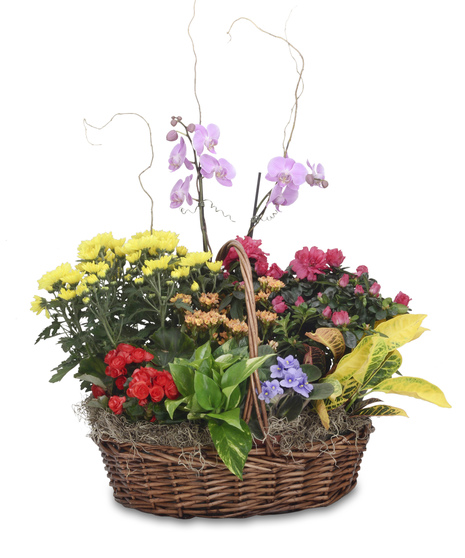This is a detailed photograph of a medium brown wicker basket with a handle, set against a solid white background. The basket, which is turned to the side in an oblong shape, is filled with a mix of vibrant and colorful flowers and foliage. The base of the arrangement consists of what appears to be dead or fake grass. 

In the forefront, to the right, green leaves and yellowish-green leaves with a touch of yellow accent occupy the lower part of the basket. To their left, a cluster of small, vibrant red flowers catches the eye. Above these, taller yellow flowers, possibly mums, are prominently displayed, and further to the left, a section of delicate, small lavender flowers balances the composition.

Towards the middle and left section, a green plant is noticeable, framed by the red flowers and supplemented by the presence of pinkish flowers. Emerging from the top, some taller features, resembling long grass with attached lavender petals, ascend, adding height and texture to the arrangement. This elegant mix of colors includes shades of yellow, pink, red, green, violet, and purple, creating a harmonious and visually appealing display.